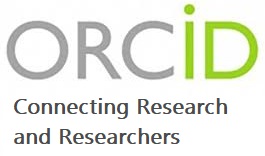The image displays a minimalist, zoomed-in section of a webpage with a plain white background. In the center, there's a sequence of text elements. The first line starts with a dark gray "ORC" in uppercase letters, followed by an "i" in lowercase, and concludes with a green "D" in uppercase. Below this, towards the center, is the phrase "Connecting Research," with both the "C" and "R" capitalized. This is followed by another centered line of text reading "and Researchers," again with the initial letters "A" and "R" capitalized. The image appears to be a close-up of a logo or branding text on a website, with no additional elements or context within the cropped boundaries of the image.